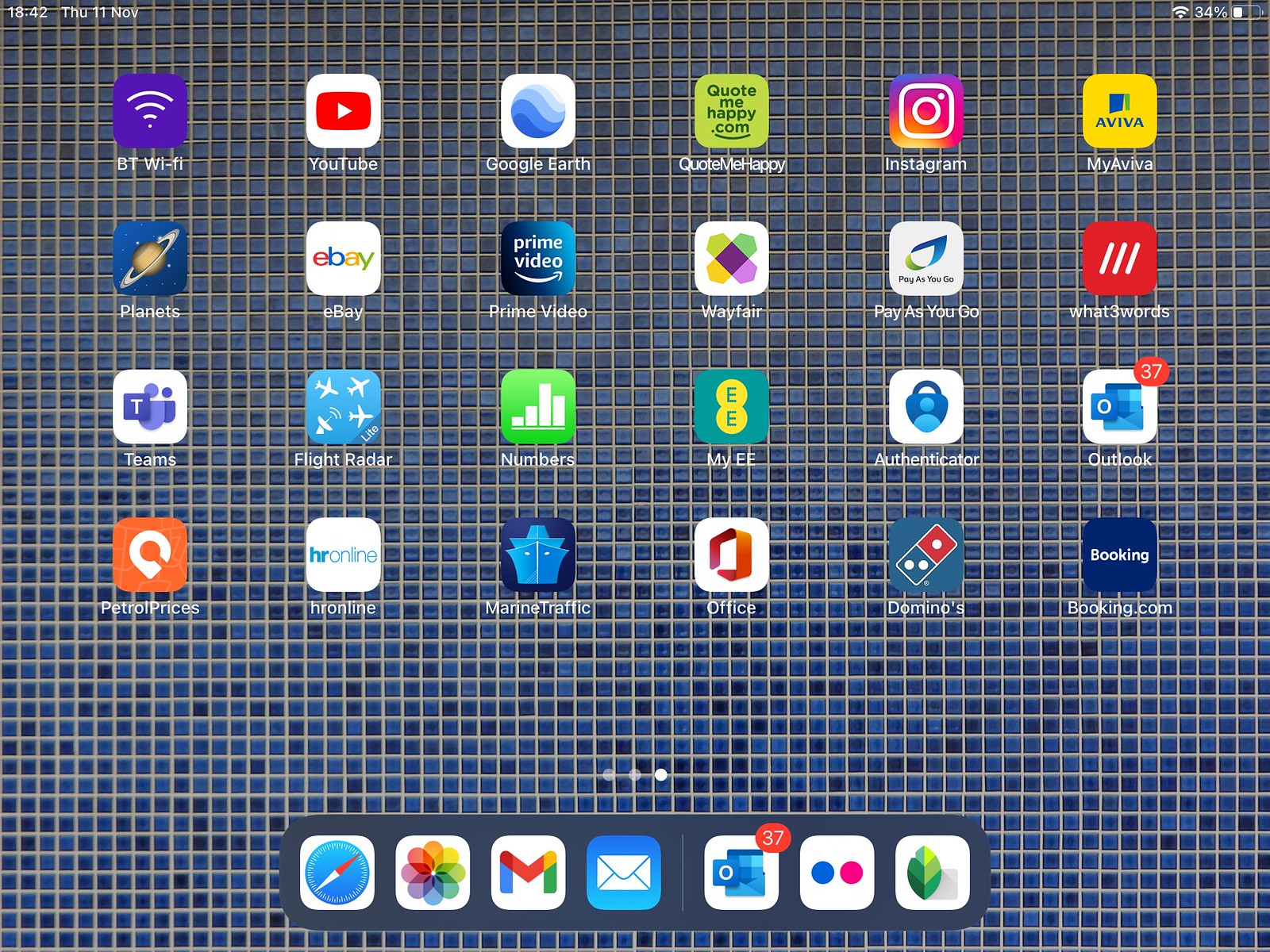The image depicts an older model desktop computer running on a Windows operating system. The desktop background features a simplistic, tiled pattern with a gradient shading from light gray at the top to darker blue at the bottom. Displayed prominently at the top of the screen, the information bar reads: "1842, Thursday, 11 November," and notes that the Wi-Fi availability is at 34%, suggesting that this might be a screenshot from someone's mobile device connected to a Wi-Fi network.

The desktop is populated with a 6x4 grid of icons, totaling 24 shortcuts. Starting from the top-left corner and moving across each row, the icons are as follows:

1. **BT Wi-Fi**
2. **YouTube App**
3. **Google Earth App**
4. **Quote Me Happy**
5. **Instagram**
6. **My Aviva**

The second row includes:
1. **Planets**
2. **eBay**
3. **Prime Video**
4. **Wayfair**
5. **Pay As You Go**
6. **What Three Words**

The third row features:
1. **Teams**
2. **Flight Radar**
3. **Numbers**
4. **My EE**
5. **Authenticator**
6. **Outlook**

The final row consists of:
1. **Petro Prices**
2. **HR Online**
3. **Marine Traffic**
4. **Office**
5. **Domino's Pizza**
6. **Booking.com**

Each icon represents a distinct application or service, catering to various tasks and interests, from productivity and online shopping to social media and navigation. This detailed snapshot provides an insightful glimpse into the user's frequently accessed applications and organizational style.